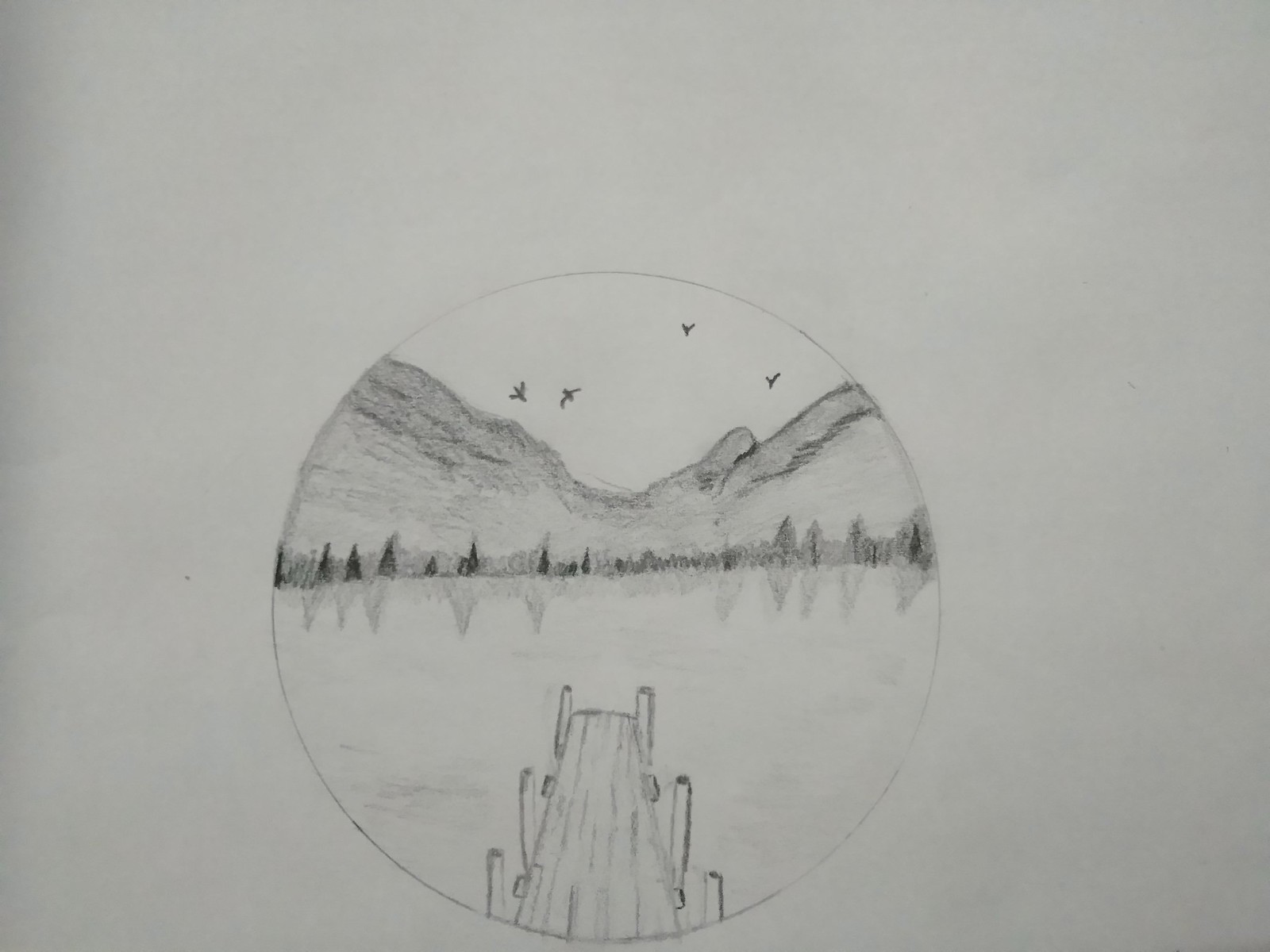This is an image of a sketchbook page featuring a detailed pencil drawing. The drawing depicts a serene lakeside scene framed within a circle that occupies about half of the page and is centered slightly towards the bottom middle. The focal point is a wooden dock with three sets of poles extending into the calm lake, which mirrors the surrounding landscape. Dense trees encircle the lake, their reflections adding depth to the tranquil water. Beyond the lake, a range of mountains rises majestically, with four birds soaring in the sky overhead. The entire composition inside the circle is carefully rendered with delicate pencil strokes, evoking a sense of simplicity and tranquility. The sketch is done on light gray paper, making the intricate details of the scene stand out distinctly.